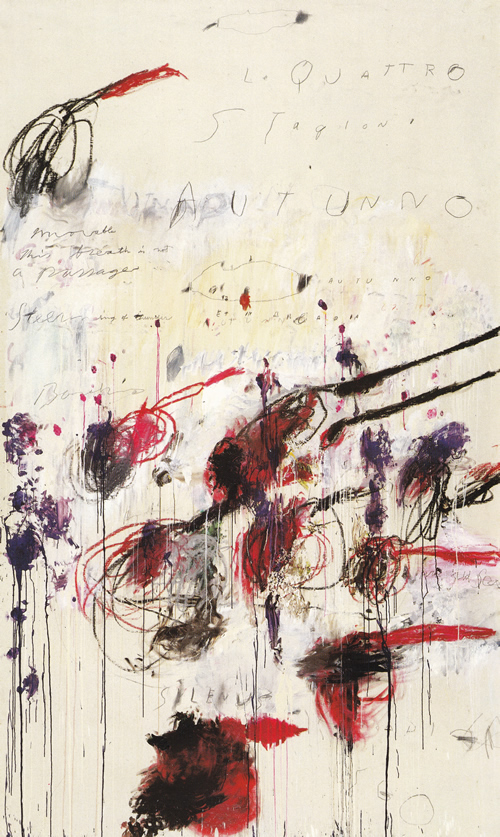This vertical rectangular image, titled "Four Seasons: Autumn" by Cy Twombly, is an intricate abstract painting on a cream-colored paper. The top of the image features a less visually cluttered area with faint pencil scribbles and a discernible crude drawing, possibly resembling a submarine. The upper left corner has faint, barely legible printed text, while the upper right shows more scribbling in various colors.

Dominating the lower two-thirds of the painting are numerous abstract figures, primarily in red and black. These figures resemble bird-like forms, each with a red chest and beak, accompanied by black wings. Surrounding these forms are vertical black lines and scattered black circles, some of which appear fuzzy or smudged, giving a sense of motion and fluidity. The red and black lines extend across the bottom portion of the image, creating a dense, dynamic composition indicative of Twombly's abstract style.